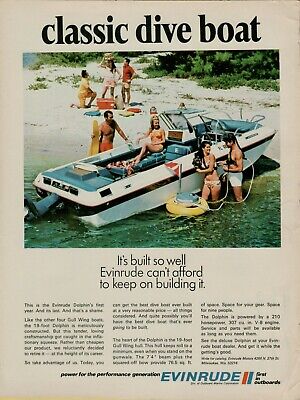This vintage advertisement, likely from the 1940s or 1950s, promotes a classic dive boat with the tagline "It's built so well, Evinrude can't afford to keep on building it." The ad features a colorful illustration in a vertical rectangle format. The primary colors are red, orange, yellow, green, blue, white, black, and beige, with "Classic Dive Boat" prominently displayed at the top. Below the text, the image shows a small, open-air speedboat with an inboard motor, finished with a white exterior and blue interior. The boat, capable of holding about eight people, is beached on a sandy shore. Around the boat, seven individuals—three men in swim trunks, four women in bikinis, and possibly an eighth person whose gender isn't clear—are either standing on the beach or in the water. Additional details include a life ring floating nearby and more people picnicking in the background. At the bottom, the ad concludes with "Power for the performance generation, Evinrude," emphasizing the boat's robust design and advanced engine.